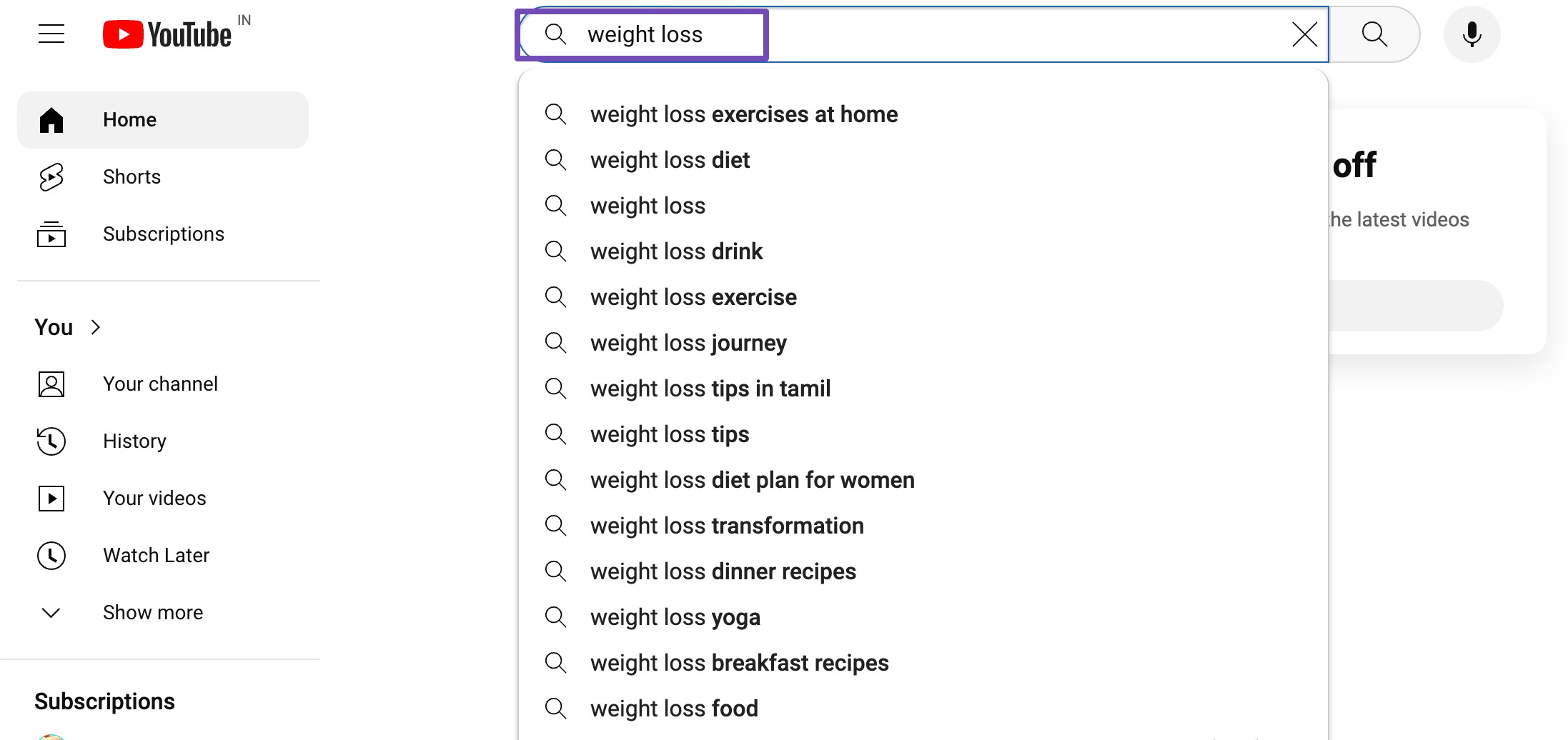The image is a screenshot of a YouTube page displayed on a desktop interface. At the top center of the image, a search query for "weight loss" is prominently enclosed in a purple rectangle, indicating it has been actively inputted. Below this primary search term, an array of suggested search variations appears, each preceded by a small magnifying glass icon. These suggestions include "weight loss exercises at home," "weight loss diet," "weight loss drink," "weight loss exercise," "weight loss journey," "weight loss tips," "weight loss meal tips," "weight loss diet plan for women," "weight loss transformation," "weight loss dinner recipes," "weight loss yoga," "weight loss breakfast recipes," and "weight loss food." Each suggested term is displayed in standard white text against the page's background.

On the left pane of the image, partially visible menu options are listed. The discernible options include "Search," "Home," "Shorts," "Subscriptions," "You," "Your channel," "History," "Your videos," "Watch later," and an option to "Show more," although the lower portion of this menu is somewhat cut off from view. This detailed layout provides a clear indication of the YouTube interface and user interaction related to the search for weight loss content.